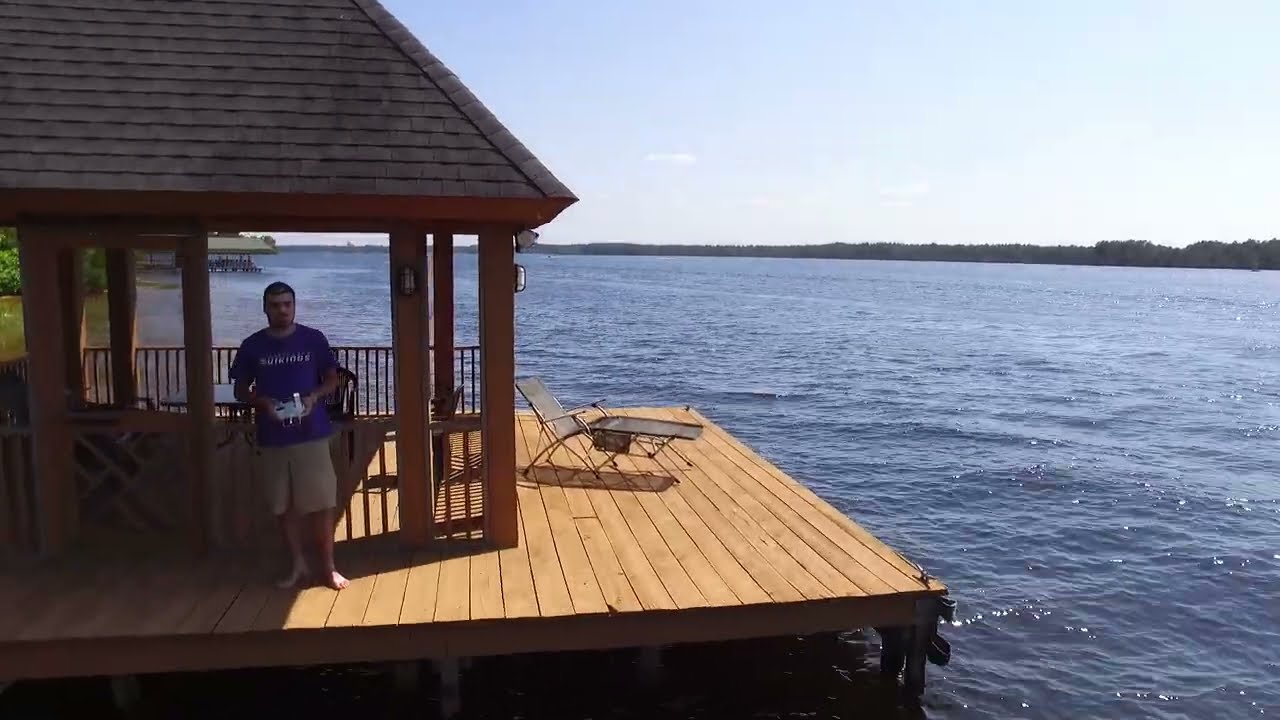The image captures a serene lakefront scene in bright daylight, likely during summer. A man stands barefoot on a tan wooden dock extending over the blue water, clad in a blue t-shirt with white writing and tan shorts. He holds what appears to be a remote control in his hands, perhaps operating a boat in the distance. Positioned under a wooden-shingled gazebo-like structure to the left, the man stands mostly in the shade, surrounded by wooden pillars. To the right, a black lounge chair sits in the sun on the dock, offering a perfect spot for relaxation. The expansive body of water is bordered by a distant tree line on the horizon, beneath a blue sky speckled with clouds. Another similar pier with a roof can be seen farther away, hinting that this idyllic setting might be part of a resort or private lakefront property.